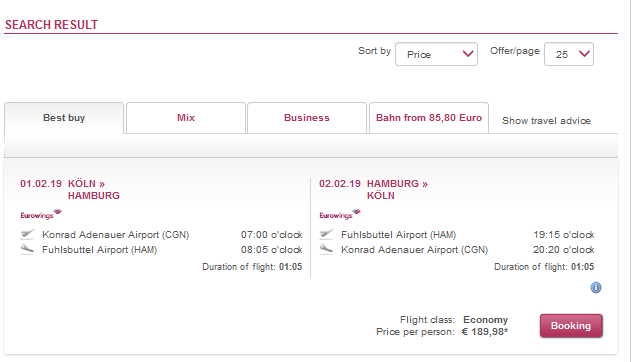This screenshot captures a web page displaying search results for flights. At the top, a header reads "Search Result" followed by a red line across the page. Towards the right, there are two drop-down menus, one labeled "Sort By" and the other with "Price" indicated inside a box, suggesting it allows for sorting options. Next to these is another drop-down labeled "Offer/Page" set to 25, enabling a different number of offers to be displayed per page.

Below this, there are four selectable tabs with "Best Buy" currently chosen. Under this tab, detailed flight information is presented. 

One of the flights listed is titled "Mix Business Bond Forum." The cost is noted as "85,80 €." Beneath it, an advisory in what appears to be German is provided: "Show Travel Advice." 

The detailed itinerary includes:
- Outbound flight on 01.02.19 from Köln (CGN), Conrad Adenauer Airport, departing at 7:00 AM, arriving in Hamburg (HAM), Fuhlsbüttel Airport, at 8:05 AM. The flight duration is 1 hour and 5 minutes, operated by Eurowings.
- Return flight on 02.02.19 from Hamburg (HAM) to Köln (CGN) with corresponding times and the same flight duration, classed as economy. 

The price per person for the round trip is 189,98 €. A prominent red button labeled "Booking" is present at the end of the listing, allowing the user to proceed with the reservation.